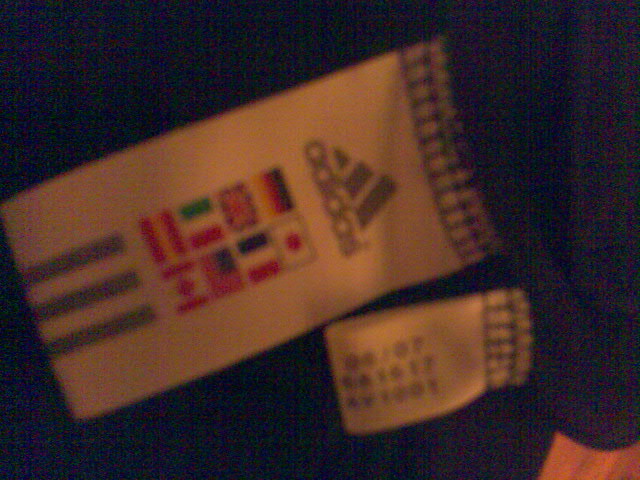The image depicts a black shirt featuring two sewn white tabs, prominently displayed. The upper tab is emblazoned with the Adidas logo, consisting of a triangular shape accompanied by two gray lines. Below this, the lower tab showcases a sequence of national flags in the following order: German, Japanese, British, black-white-red tricolor, Italian, American, Spanish, and Canadian. The bottom left corner of the tab displays alternating blue and white lines, while the bottom right corner contains some indistinct text. The overall image appears slightly out of focus, with a grainy texture adding to the blurriness, especially noticeable in the bottom right section where there’s a brownish hue.